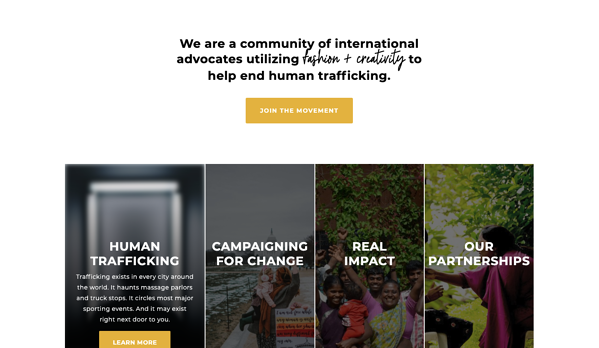The image features a visually striking advertisement for a community dedicated to fighting human trafficking through fashion and creativity. At the top, a meaningful message in elegant black cursive text reads, "We are a community of international advocates utilizing fashion and creativity to help end human trafficking." Below this, a bold yellow horizontal box with white text encourages viewers to "Join the movement."

Further down, various interactive options are presented. The first option, "Human Trafficking," is highlighted in bold white text. There is also a clickable yellow box labeled "Learn More," prompting deeper engagement. This section is followed by "Campaigning for Change," presented in clean white text.

The section titled "Real Impact" includes an uplifting image of a diverse group of individuals smiling joyfully, with their hands raised in the air, set against the backdrop of a large, lush tree. Finally, the map directs attention to "Our Partnerships," emphasized with uppercase bold white text. Accompanying this is an image of a person adorned in a vibrant pink garment, standing before tall, verdant green trees, visually capturing the essence of collaboration and natural beauty.